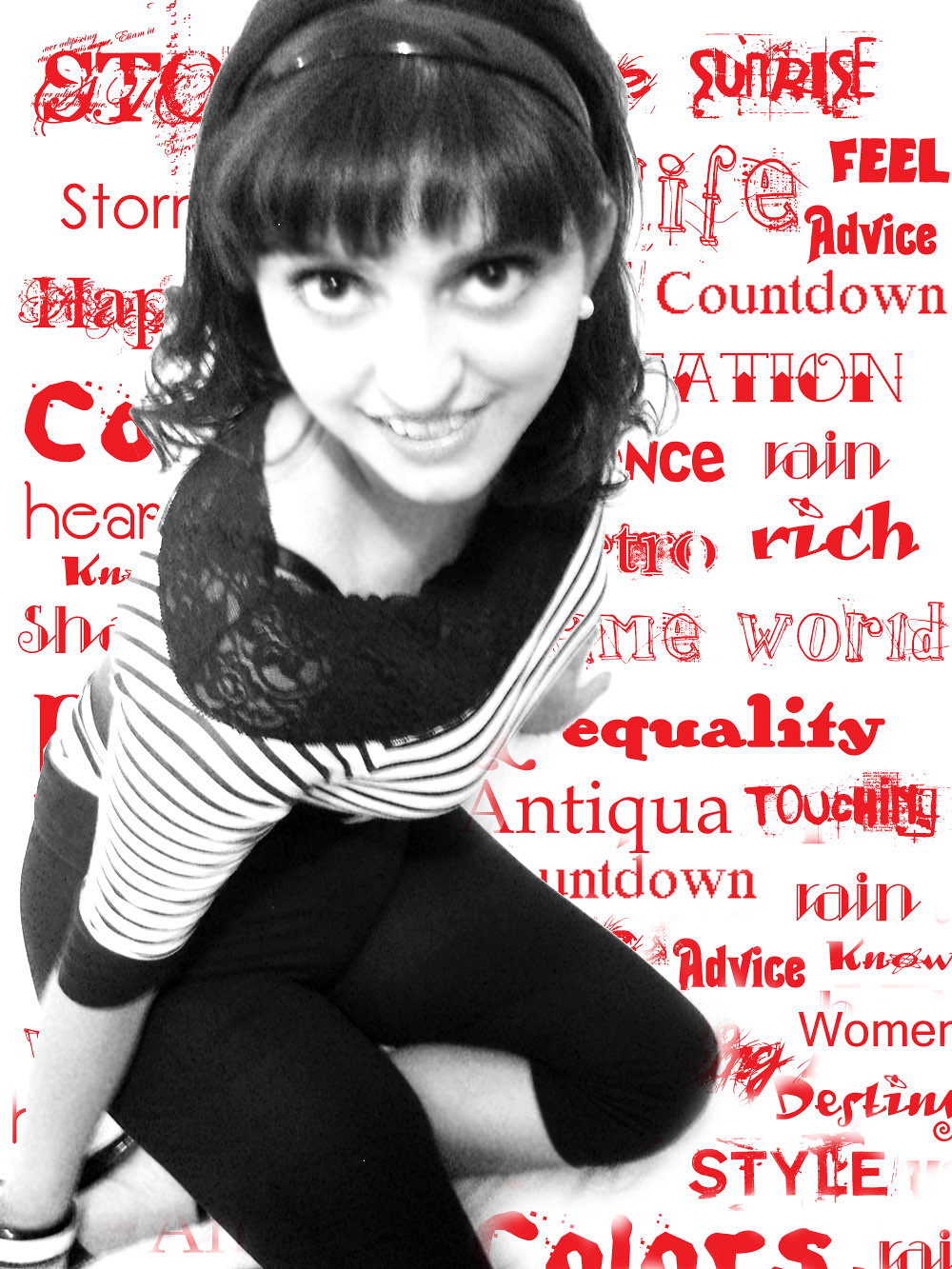The image features a young woman depicted in black and white. She has short, dark hair styled with bangs that fall just above her eyebrows, and she's adorned with a dark-colored plastic headband. Her hair reaches her shoulders and is flipped outward, complemented by pearl earrings and a black and white bracelet. She is dressed in knee-length black pants and a boat-neck striped top with a lace collar. The woman, thin and smiling, is kneeling on the ground, possibly sitting on a bed or couch, and appears to be bent slightly at the waist as she looks upward towards the camera.

The background is white and filled with numerous red words in various edgy fonts. Some of the discernible words include "feel," "advice," "countdown," "nation," "rain," "rich," "world," "equality," "antiqua," "women," "design," "style," and "destiny." The scattered text partially obscured by her presence, adds a visually dynamic and textured backdrop to the composition.